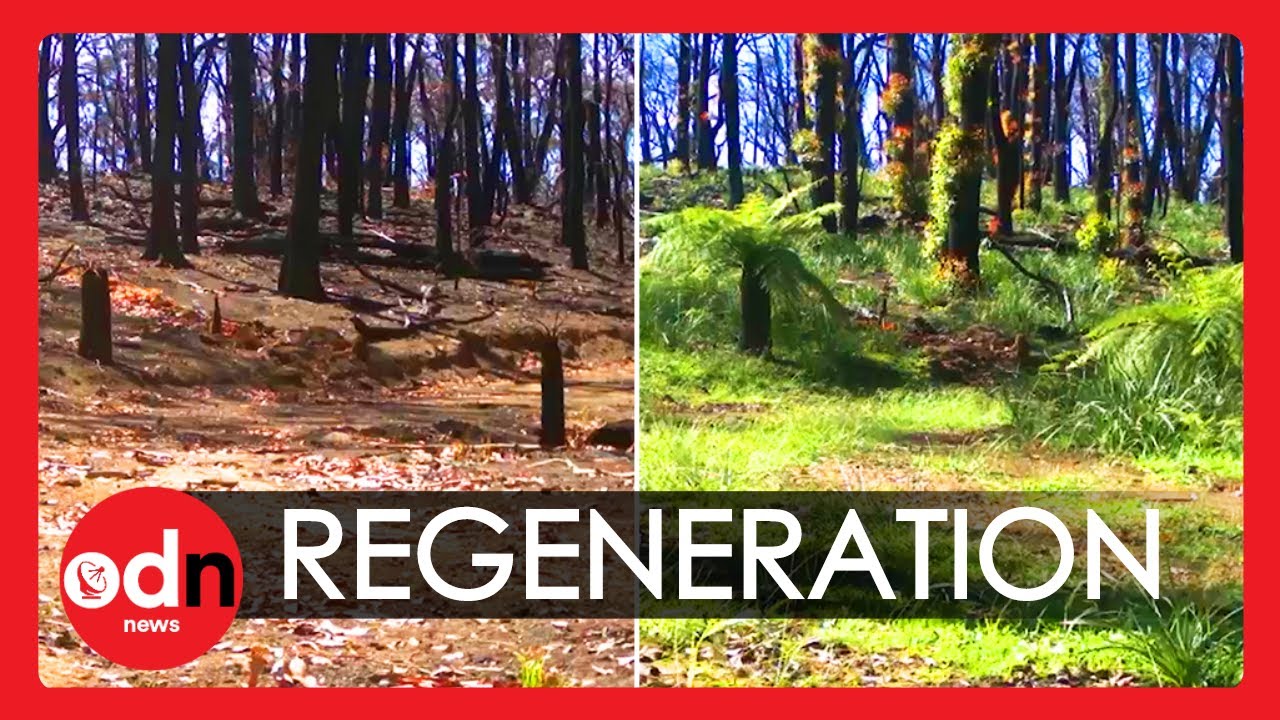The image, framed by a red border, consists of two side-by-side photos showing a forest landscape transitioning from devastation to renewal. The left photo captures a scorched forest aftermath, with barren ground strewn with red dead leaves and trees stripped of foliage, some visibly fallen or broken near their bases. The charred black trunks and erosion dominate the scene, suggesting the forest was badly burned, potentially due to a fire.

The right photo offers a striking contrast, depicting the same forest area rejuvenated. Lush greenery has sprung up, with moss and vines covering the once-scorched trees. The forest floor is now covered with vibrant green plants, and trunks that were once blackened now showcase signs of life and growth. There are also various plants, some even with reddish hues, winding around the trunks. The blue sky visible through the trees in both photos highlights the passage of time and nature’s resilience.

The bottom of the image is overlaid with a semi-transparent black banner displaying the word "regeneration" in white text, indicating the theme of the transition shown. In the lower left corner, the logo “DN News” is marked within a red circle, signifying the source of the visual story.